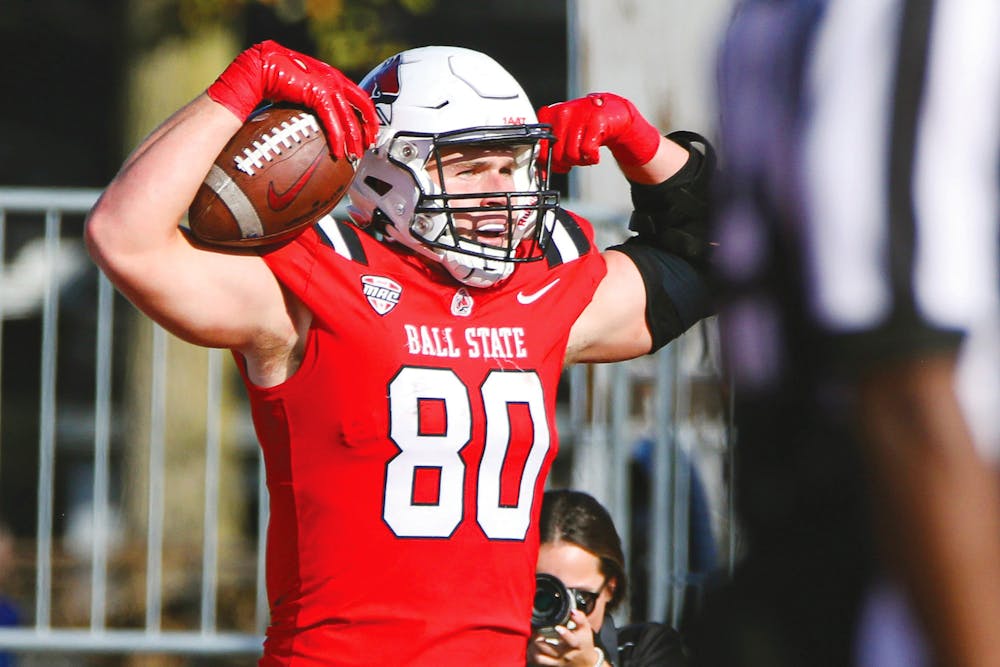A college football player from Ball State, sporting the number 80 jersey, stands prominently at the center of the image. He is outfitted in a striking red uniform with white and black accents, including the bold white "Ball State" lettering and prominent number 80 on his chest. His red gloves, shiny and leather-like, grip a brown football with a red Nike emblem in his right hand, while his left hand is raised up by his white helmet, which features a detailed red cardinal logo with a white beak and black stripe. The player looks intensely ahead, his mouth open, possibly mid-celebration after a successful play. His left arm is adorned with an elbow guard. In the background, a blurred referee's shoulder and hand in a white and black uniform can be seen to the left, and to the right, a woman kneels with a camera, capturing the moment, her dark hair visible. Behind them, a white fence and some greenery further frame the scene.